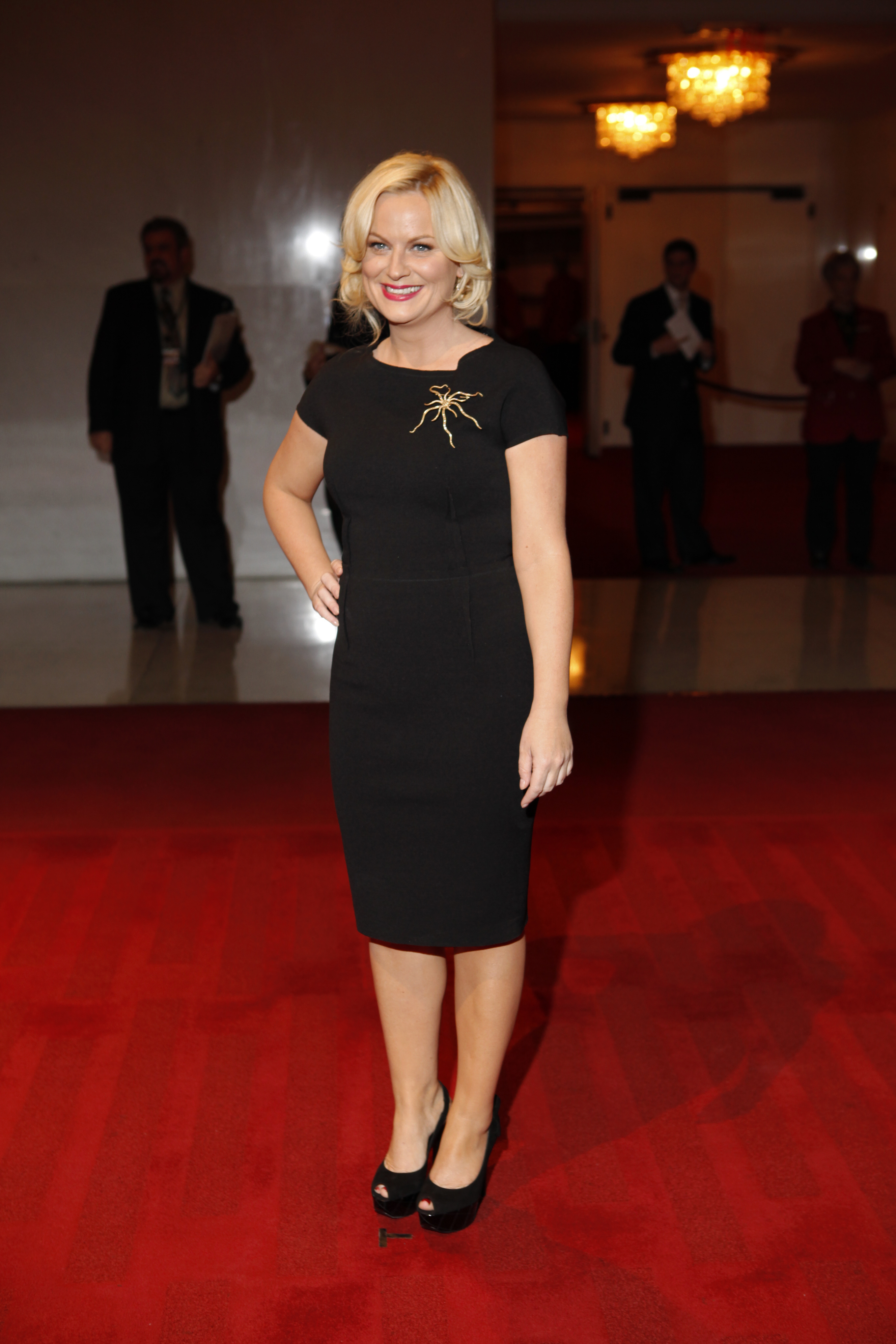In this image, Amy Poehler is standing and posing on a glowing, lit red carpet, likely in a ballroom, event center, or hotel lobby setting. The scene is characterized by hardwood and tile floors, chandeliers, and open doors. Amy, a middle-aged woman with medium-length blonde hair and blue eyes, is wearing a black dress with short sleeves, black high heels, and a gold accent adorning the right side of her chest. Her makeup includes bright red lipstick, and she has her right arm on her hip, smiling directly at the camera. Surrounding her are five people in suits and ties, likely ushers or attendants, with two men positioned to the right in front of a door, another man by the wall to the left, and more individuals dispersed in the background. The overall color palette includes burgundy, red, black, white, tan, blonde, and glowing yellow, contributing to the event's vibrant atmosphere.